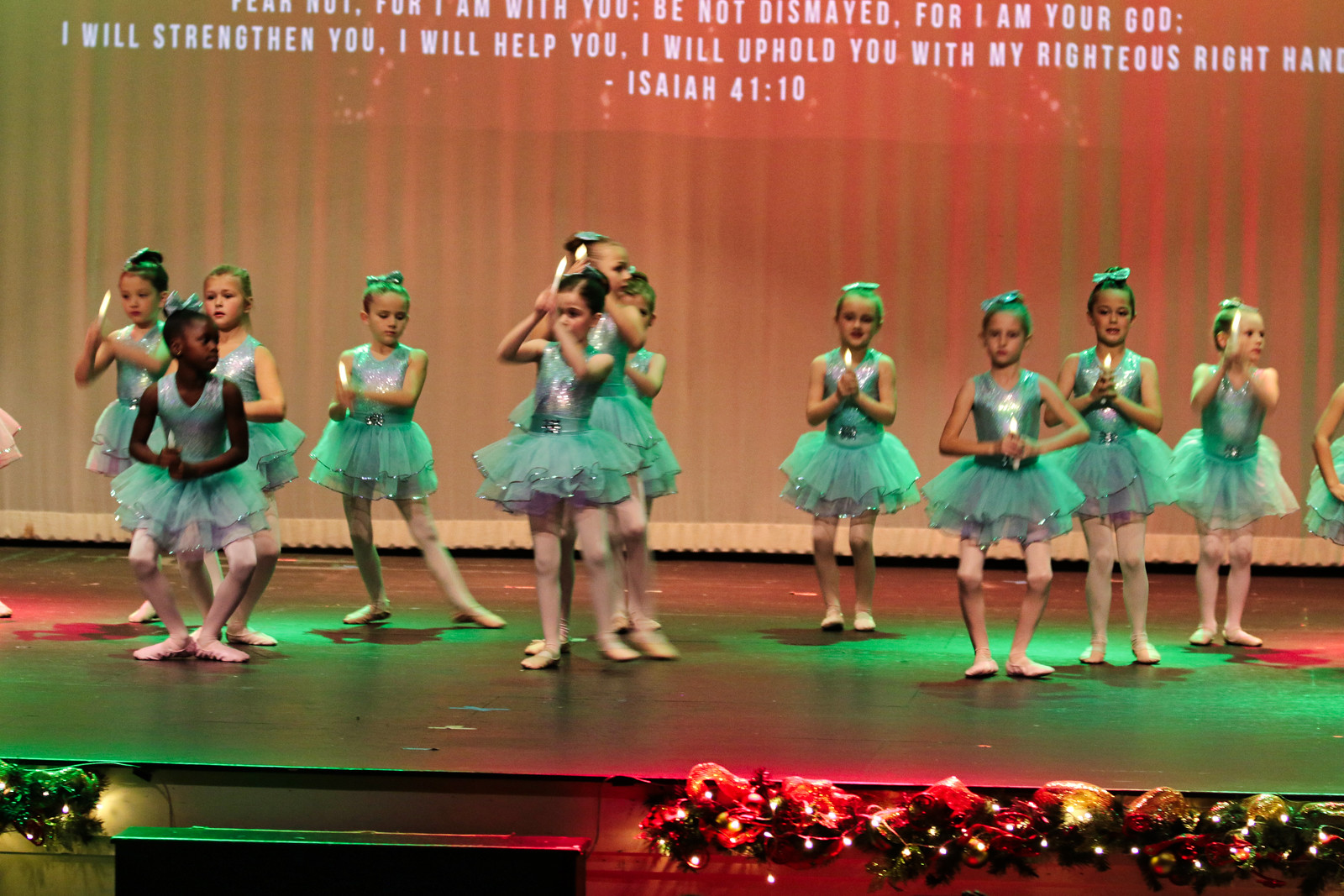The photograph captures a holiday-themed, religious ballet recital featuring eleven young girls, likely around five years old, on a well-lit stage. The girls are dressed uniformly in silvery-gray leotards with tulle skirts, complemented by tights and ballet shoes, and they are in the midst of a dance. Each girl holds a battery-operated candle, enhancing the festive atmosphere. The stage is adorned with green and red lights, both projected onto the scrim behind the dancers and illuminating the performance area. Christmas decorations, including lighted greenery and cedar wreaths with red ribbons, are draped along the bottom front edge of the stage, adding to the seasonal ambiance. Above the performers, white text displays a biblical verse: "Fear not, for I am with you. Be not dismayed, for I am your God. I will strengthen you. I will help you. I will uphold you with my righteous right hand. Isaiah 41:10." The audience's perspective of the photograph captures the joy and significance of this heartfelt holiday performance.